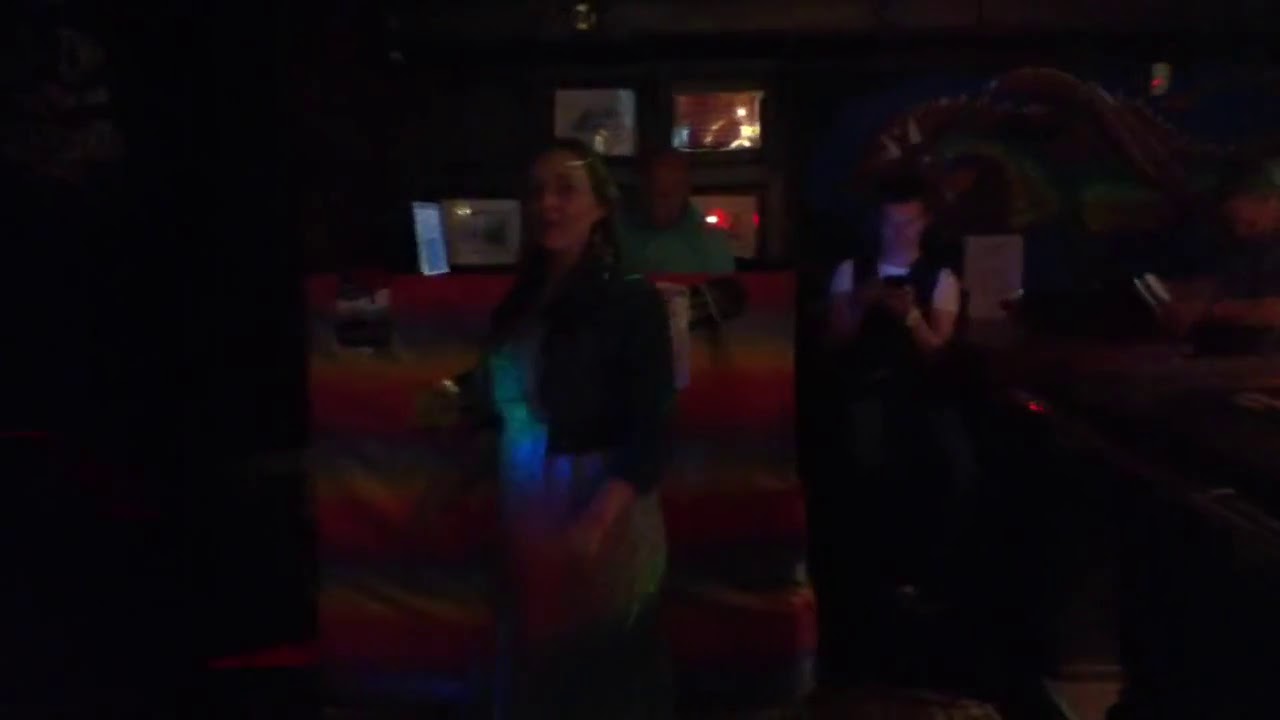In a very dark and blurry room, a middle-aged woman is at the forefront, capturing attention with her long straight dark hair. She wears a green dress possibly paired with a blue jacket, standing in front of a vividly colorful, rainbow-striped blanket or backdrop. Despite the dim lighting, her face is directed towards the camera. Behind her, an older bald man in a light green shirt is partially visible, and next to him is another man wearing a black vest over a white shirt, intently focused on a phone or writing something down. The background is adorned with shiny framed photos, though the darkness obscures further details, giving the entire scene a hazy and indistinct ambiance.